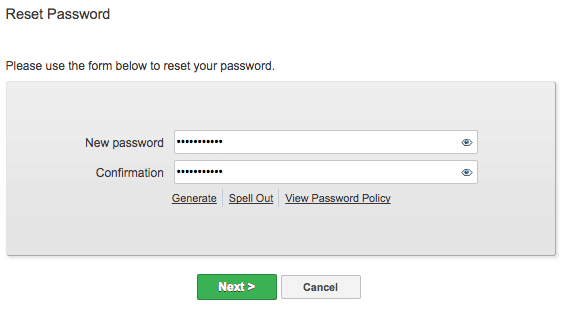The image depicts a password reset screen, partially cropped, making it unclear which website or app it belongs to. At the top, in bold text, it reads "Reset Password," followed by smaller text instructing, "Please use the form below to reset your password." The form is set against a gray background within a rectangular box.

The first field is labeled "New Password" and contains a white input box where the password is obscured by black dots, indicating hidden text. Adjacent to this field is an 'eye' icon with a blue iris, which likely allows the password to be revealed when clicked. Below this, a second field labeled "Confirm Password" mirrors the first, with hidden text represented by black dots and another identical 'eye' icon.

Below the input fields, there are three underlined and clickable text options: "Generate," "Spell out," and "View Password Policy," each in black text. At the bottom of the form, there are two buttons: a green "Next" button with white text and a black "Cancel" button, both rectangular in shape.

The form's container is set against a white overall background, contrasting the gray section dedicated to the password inputting process, ensuring users can distinguish the interactive elements easily.